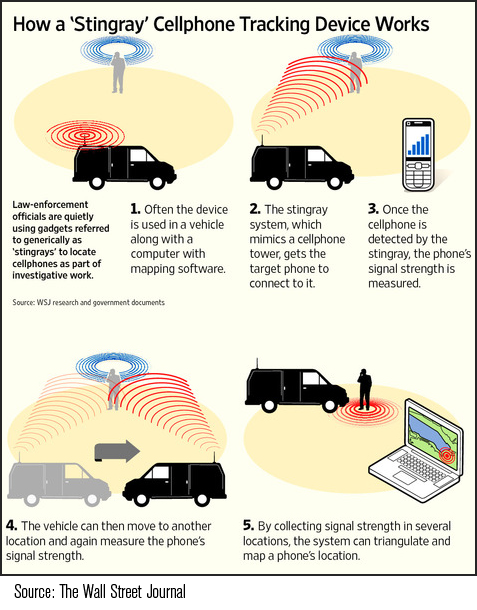The image, sourced from The Wall Street Journal, is an infographic titled "How a Stingray Cell Phone Tracking Device Works," set against a pale yellow background bordered with a thin black line. It details the process in five illustrated steps, each depicting a black panel van equipped with an antenna, emitting red rays toward a target. 

1. The first illustration shows the van emitting rays towards a gray silhouette of a man highlighted with a blue outline.
2. In the next image, the rays target both the man and an illustration of a cell phone.
3. The third image depicts two vans facing each other, both emitting rays towards the man.
4. The fourth step shows the van in close proximity to the man, emitting red rays while the man, now black, has no blue outline, indicating a connection.
5. A nearby open laptop is shown, symbolizing the data collection.

The accompanying text explains that law enforcement officials are using these Stingray devices, which mimic cell phone towers to trick target phones into connecting. The system then measures the phone's signal strength to triangulate its location by moving the van and collecting data from various points. The information in the infographic is corroborated by WSJ research and government documents.